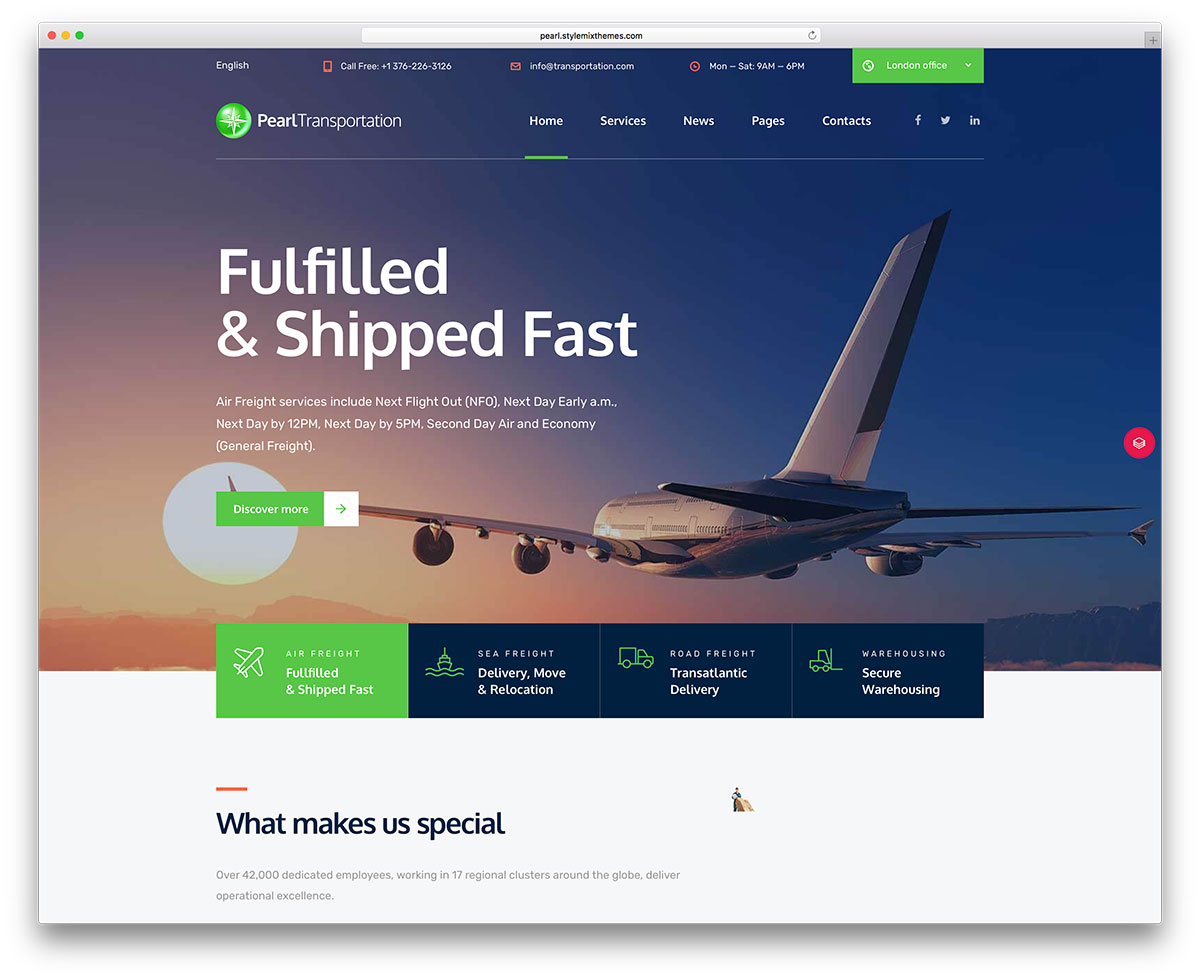In the upper left corner of the image, a website is displayed within a browser that closely resembles Safari. The URL bar shows an address starting with "Wetabyte," although the complete details are unclear due to the smaller image size. At the top of the website, there's a navigation section with options for language selection (English), a call prompt with a phone number, an email address, and operational hours listed as Monday through Saturday, 9 a.m. to 6 p.m. Next to this information, there is a blue button labeled "London office" featuring a globe icon and a down arrow, followed by a lighter, neon green button.

Below these navigation options, the company logo is visible. The logo appears to be a stylized star, reminiscent of a light glare with varying axes, overlaid on a 2D surface resembling a globe, all in different neon green shades. To the immediate right of the logo, the website menu includes links to sections such as Home, Services, News, Pages, and Contacts, along with social media icons for Facebook, Twitter (or X), and LinkedIn.

Further down, the page highlights a promotional message: "Filled and shipped fast, air freight service includes next day, or next flight out, next day early A.M., next day by 12 p.m., next day by 5 p.m., second day air and economy general freight." There is a "Discover more" button accompanied by an image of an airplane in flight with the sun positioned to the plane's left and part of the horizon visible at the bottom of the image.

At the bottom of the webpage, there are various sections labeled Air Freight, Sea Freight, Road Freight, and an unreadable last section. A segment titled "What Makes It Special" is featured further down.